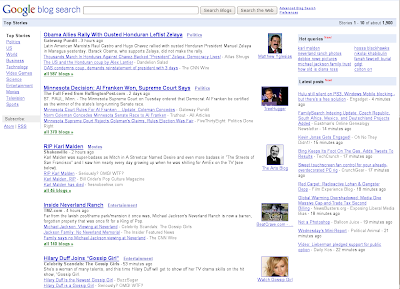This is a small and barely legible screenshot of a Google search page. Prominently at the top left is the distinctive Google logo, featuring a blue "G," red "O," yellow "O," blue "G," green "L," and red "E." Below the logo, the words "Blog search" are displayed in blue. The central area of the screenshot contains a white search bar flanked by two gray buttons on its right. 

To the left of the search bar is a sidebar filled with blue links, while the main section in the center displays five search results. Each search result is highlighted with bold blue links. Adjacent to these search results, there are five small images positioned either to their left or right, but their exact placement is unclear due to the small size of the screenshot.